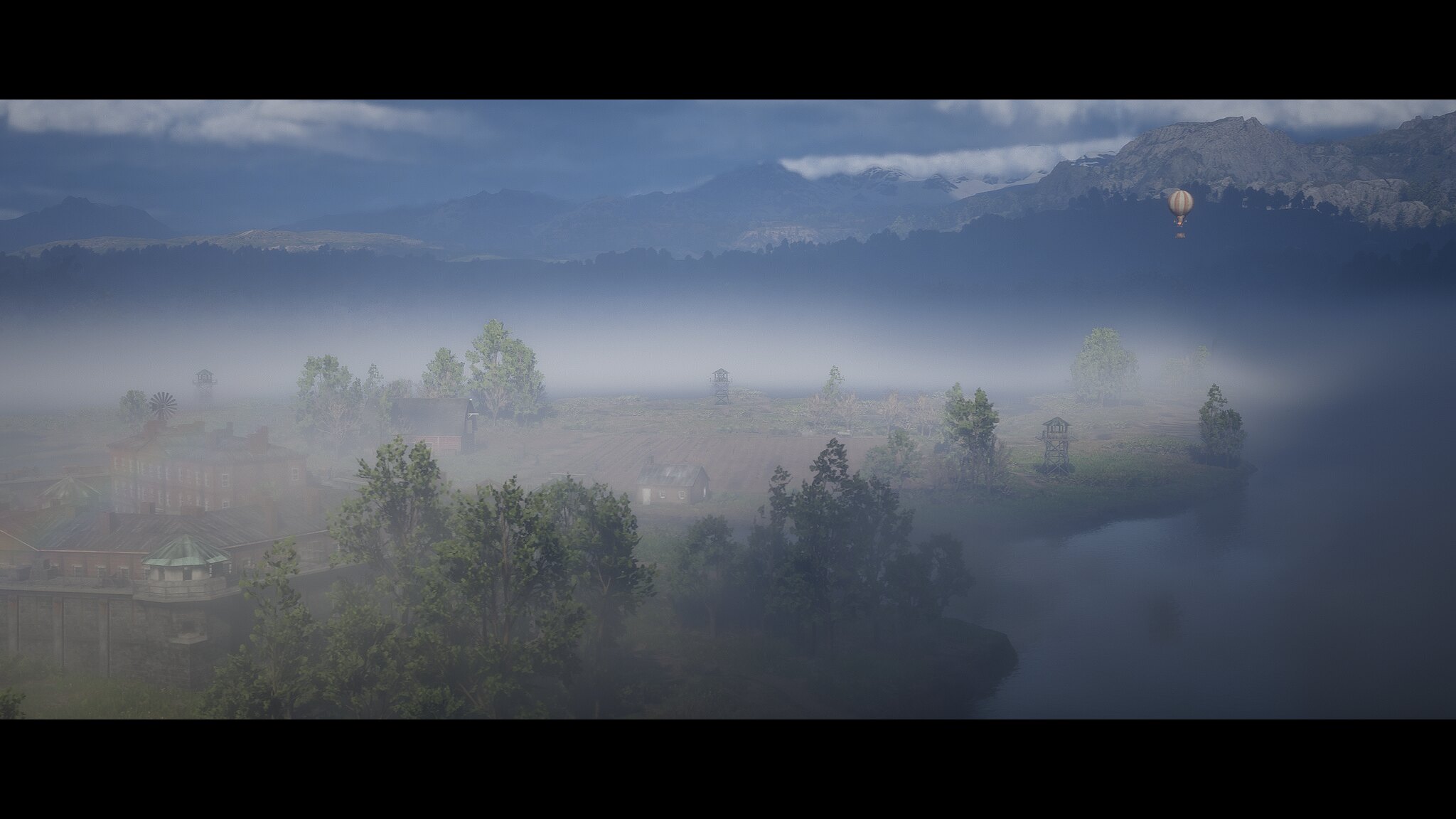The image captures a broad, foggy outdoor scene, seemingly from a movie, that stretches about 1.5 to twice as wide as it is tall. The top 10-15% of the image is letterboxed with black bars, creating a cinematic feel. The scene, likely photographed from a height akin to a drone's perspective, reveals a diverse landscape.

To the left, expansive land is dotted with sparse trees, their green foliage contrasting with the brownish terrain, which occupies about 75-80% of the image. Nestled in this area is an old concrete structure, possibly a fort, with a triangular peak visible in the lower left-hand quadrant. This side also showcases tall, bushy trees and dense greenery interspersed with patches of open, dirt-covered spaces.

On the right, a body of water, likely a lake, extends to the edge of the frame. The sky above is heavy with thick, white clouds and a dense fog or smog that blankets the entire scene. Dominating the upper right-hand quadrant, a distant hot air balloon, sporting red and white stripes, floats high in the cloudy sky. The backdrop is framed by towering mountains, enhancing the dramatic and picturesque quality of this atmospheric countryside vista.